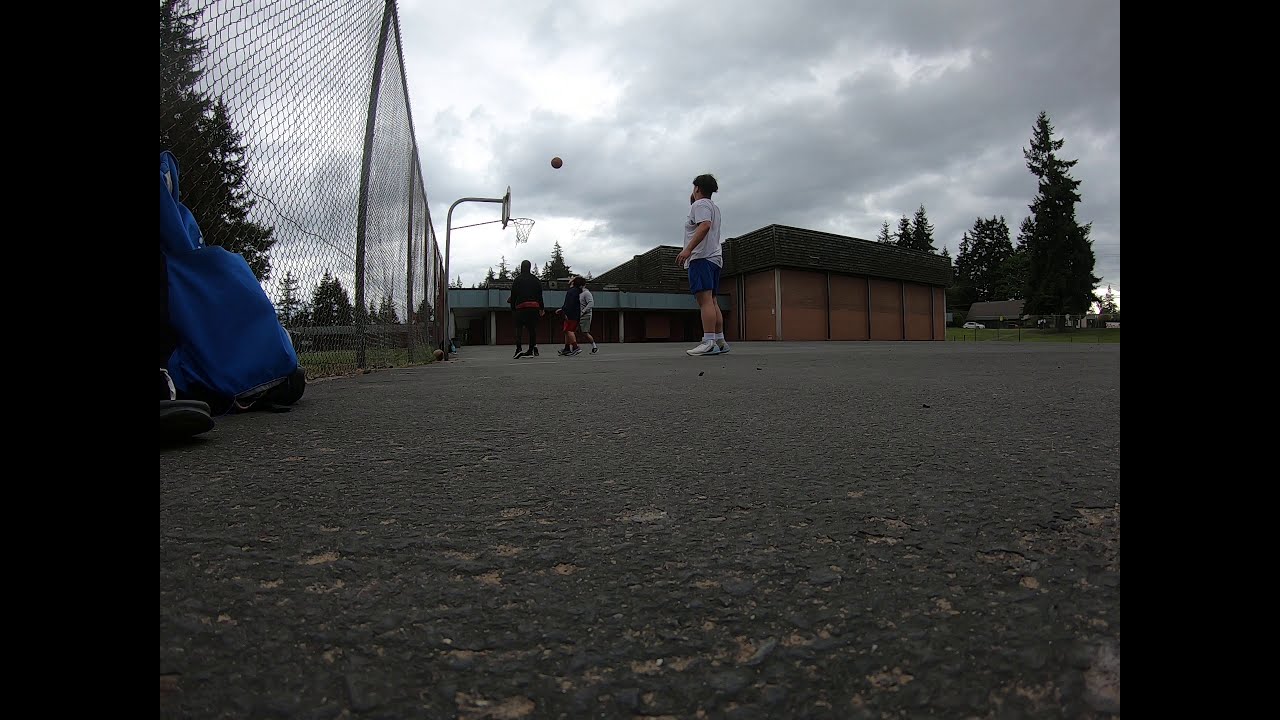In this horizontally aligned rectangular picture, taken from ground level outdoors on a cloudy, overcast day, four guys are playing street basketball. The composition suggests the camera is placed low to the ground, likely on a cracked, gray and black concrete pavement. The sky above is filled with dark gray and white clouds, with some brightness trying to peek through.

In the center of the image, the basketball is captured mid-air, about to go into the basket. Surrounding the basket are three players: two wearing black attire, one with red shorts and the other in black pants, and the third player sporting a white or gray shirt with gray shorts. Another individual stands off to the right side, dressed in a white t-shirt, blue shorts, and white tennis shoes, with short brown hair.

In the background, a one-story, windowless brown building with a dark brown roof is visible, accompanied by tall green trees partially obscuring another structure to the right. To the left of the image, a tall chain-link fence stretches upwards, with shoes peeking out at its base, suggesting someone is seated against it. More trees can be seen beyond the fence, adding to the outdoor, park-like setting.

The image exudes a casual, recreational atmosphere, with the boys seemingly enjoying a friendly game of basketball in what could be a schoolyard, park, or residential area.